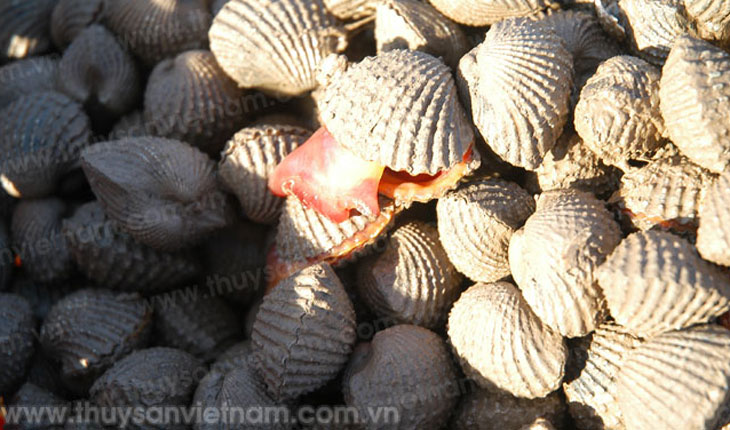This photograph captures a close-up of dozens of seashells in an outdoor setting, beautifully arranged in a horizontally aligned rectangular frame. The shells are predominantly gray, some appearing in the shadow on the left side of the image, while others bask in bright sunlight on the right, creating a distinct contrast. Each shell is textured with ridges and vertical lines, adding a tactile dimension to the scene. One shell stands out, partially open with a shiny pink body protruding, reflecting the intense sunlight. Subtle watermarks of the website www.thuysanvietnam.com.vn are visible throughout the image, more discernible on the shadowed side but less so on the brightly lit shells. The website is prominently marked in the lower left corner, suggesting an advertisement for a Vietnamese seafood or tourism site.